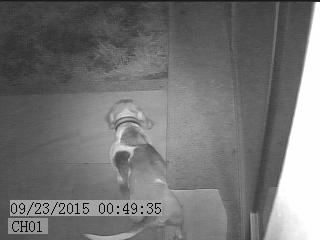Captured by a porch security camera in black-and-white, this image from the night of 09/23/2015 at 00:49:35 (CH01) shows a small dog, possibly a beagle, walking down the porch steps towards a grassy yard. The dog, positioned centrally in the image, has a collar and visible patches on its back, adding some texture to its monochromatic silhouette. The porch's structure lines the right side of the frame, identified by a white doorframe extending from the top right corner to the bottom right. Additionally, a bit of tall grass is visible beyond the porch, mingling with the shorter grass of the yard. The scene is illuminated in varying shades of gray, with no other colors due to the camera's night mode, creating an almost serene, albeit slightly eerie atmosphere. Finally, the timestamp is marked in a gray box at the bottom left, providing the exact date and time of the image capture.